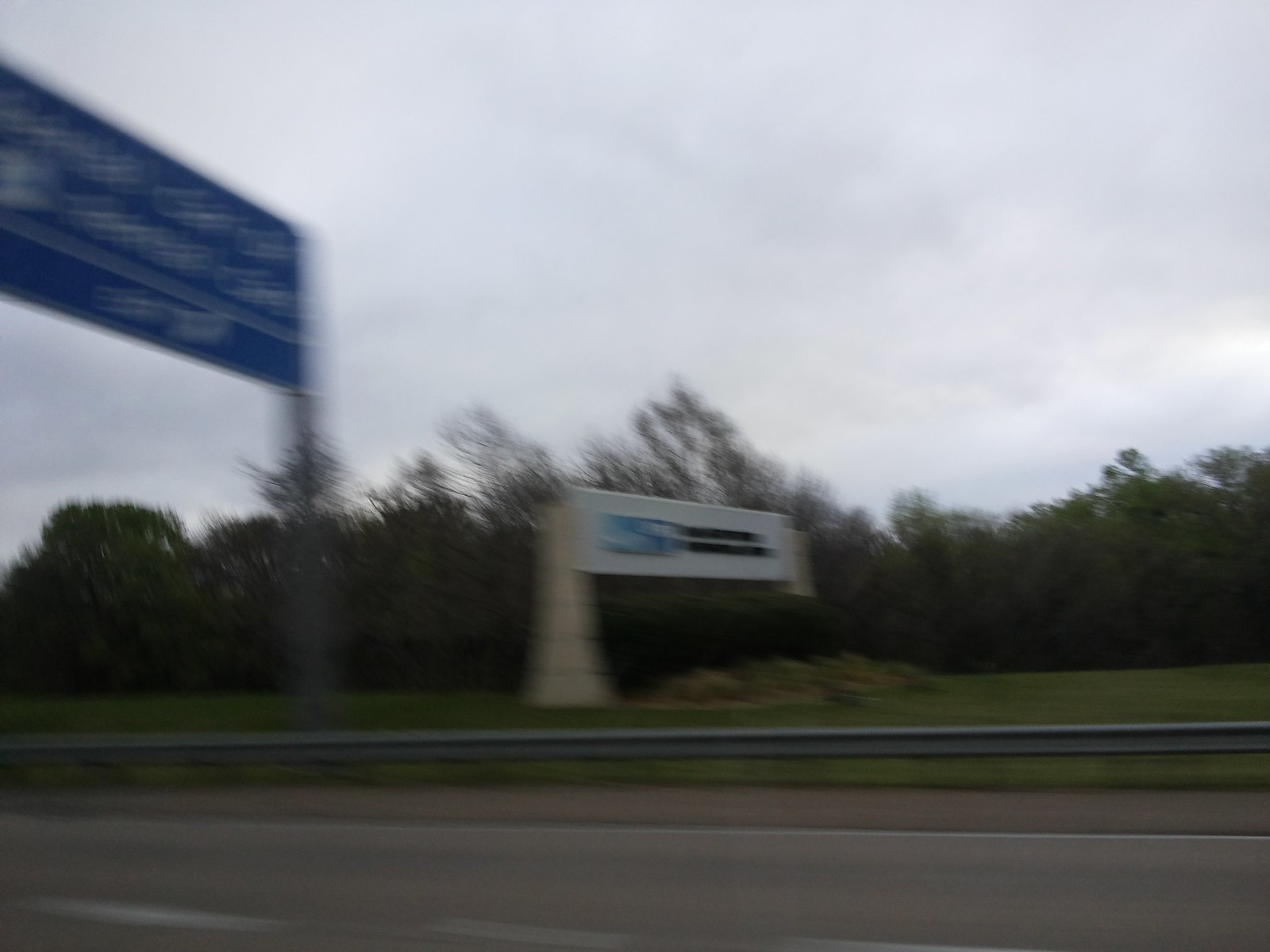A photograph captured from a moving car showcases a multi-lane road. The image frames a narrow emergency lane on the right-hand side, bordered by a white dotted line marking the adjacent lane. Prominently featured is a large sign elevated on white stands; the sign itself is white with a blue logo and black lettering, though the text is obscured by the blur from passing trees. The backdrop suggests late fall or winter with a white, cloud-filled sky. Additionally, there is an overhead blue information sign, typical of interstate or highway notifications in the United States. The exact content of the signage remains unclear due to the motion and angle of the shot.